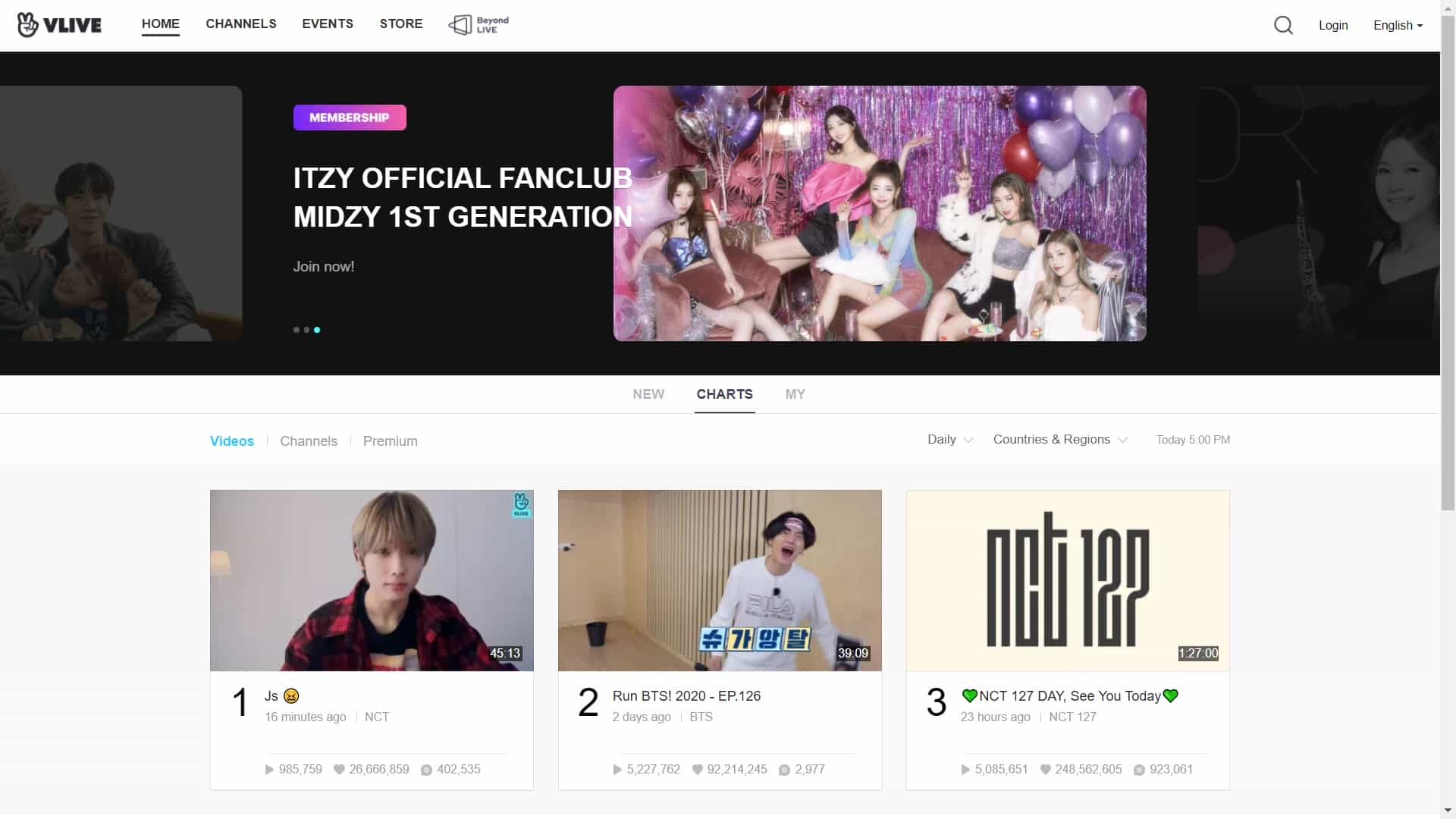At the top of the image, a white banner with black text spans across. On the left side of this banner, an outlined figure making a peace sign accompanies the "VLIVE" logo. Adjacent to it, bold black text lists navigation options: "HOME" with a black bar beneath it, followed by "CHANNEL," "EVENTS," "STORE," and "BEYOND LIVE," the latter paired with a distinctive logo.

On the right side of the banner, icons and text offer site functionalities: a magnifying glass symbol for search, "LOGIN," "ENGLISH," and a black bar. Below this bar on the left, a partially visible image suggests a person sitting. Adjacent, a purple bubble with white text reads "MEMBERSHIP." Continuing on the black bar, white text announces "ITZY" and "ITZY Official Fan Club, MIDZY's first generation."

Below the banners, a staged photograph features an ensemble of Asian women in a celebratory setting, adorned in stylish, revealing outfits, and surrounded by pink, red, and white balloons. Beneath this main image, three smaller pictures are labeled with numbers 1, 2, and 3, connected to BTS or another prominent K-pop group, suggesting the site serves as a vlog platform for K-pop enthusiasts.